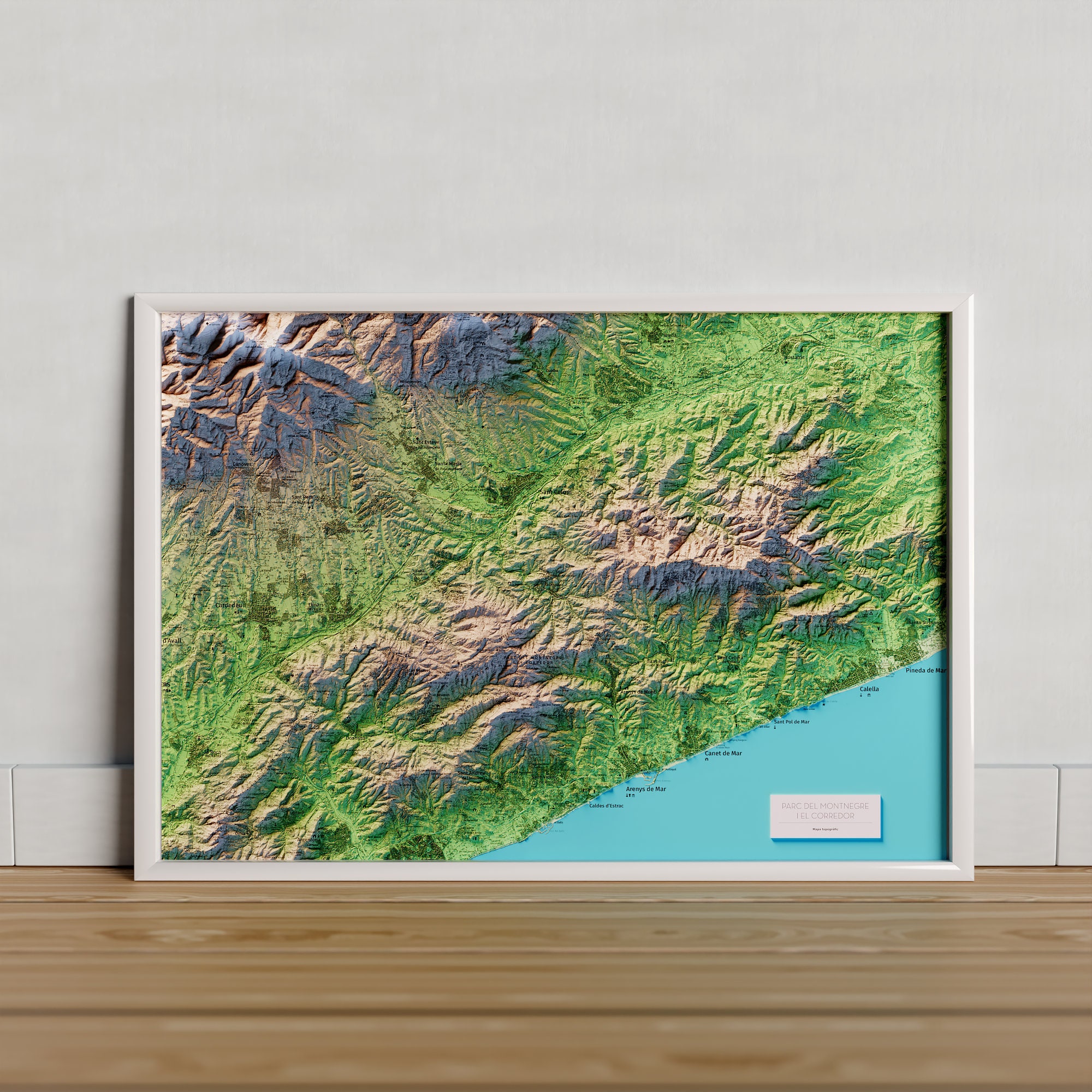The image depicts an indoor scene in what appears to be a residential room with light gray walls and a hardwood floor with light brown tones interspersed with dark wood grain patterns. On the floor, leaning against the wall, is a large, light gray frame containing a detailed map. The map shows a coastline and various land elevations with a color scheme that includes light brown, white, green, ocean blue, and gray. The map seems to portray topographical features, possibly at a regional scale, with different colors indicating various elevations. While there is some text on the map and a potential title in the bottom-right area, it is too small and blurry to be clearly legible, appearing in a very light gray font on a similarly colored background. This adds to the meticulously captured yet somewhat abstract ambiance of the artwork.